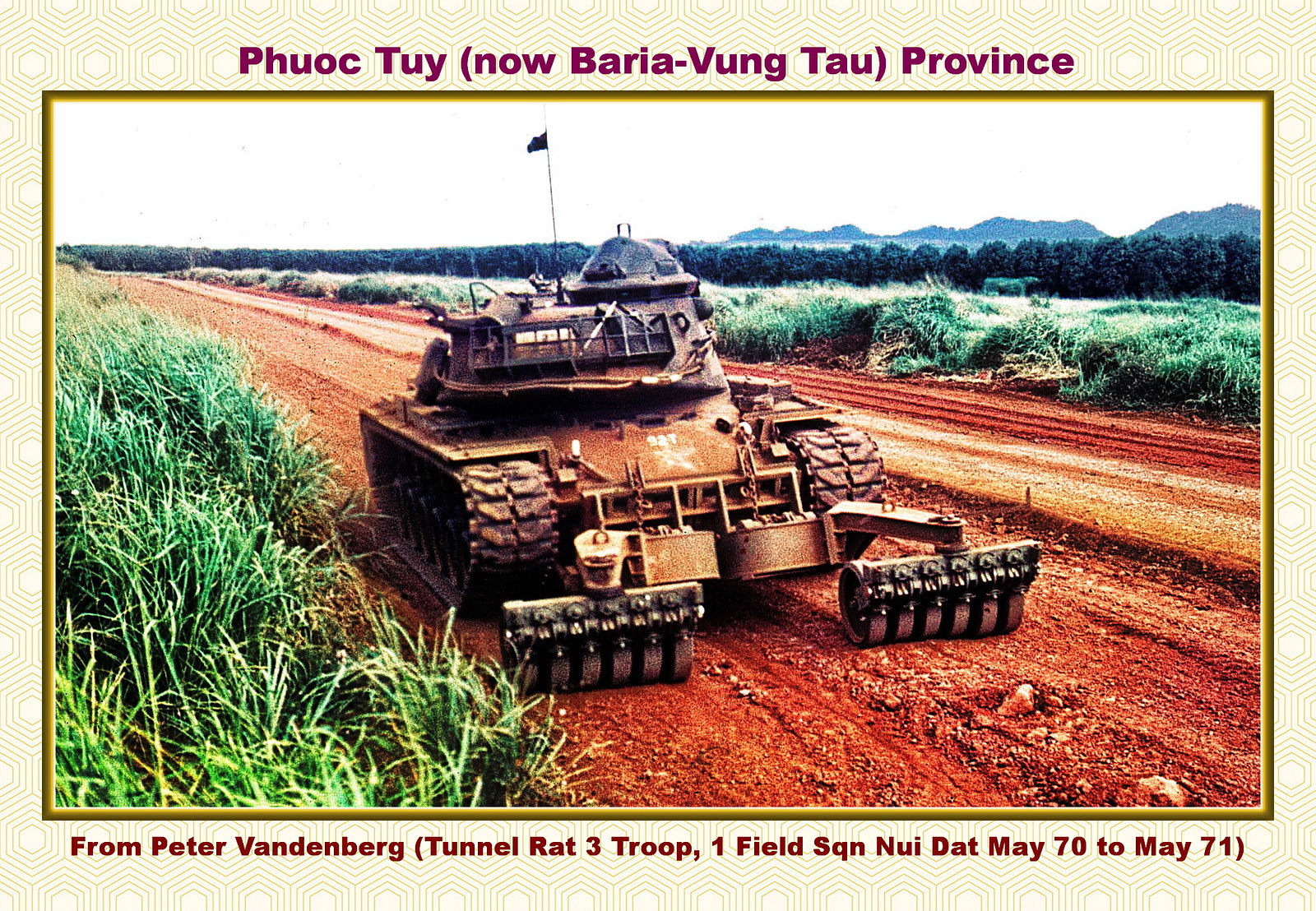This image is a detailed photograph framed by a yellow border adorned with geometric shapes. At the top of the frame, there is a purple header that reads: "Phuoc Tuy (now Baria Vung Tau province)." In the center, the photograph displays a military tank with distinctive features, including rollers on each side and two protrusions at the front, possibly for grading the ground. The tank is traveling on a red clay dirt road, slightly tilted to the right. Flag protruding from its top and a star emblem on its front plate are visible. Surrounding the road are lush green shrubbery and tall grasses, with rolling hills and trees in the distance. The bottom of the frame features a tagline in red letters: "From Peter Vandenberg (Tunnel Rat 3 Troop 1 Field SQN, Nui Dat, May 1970 to May 1971)."